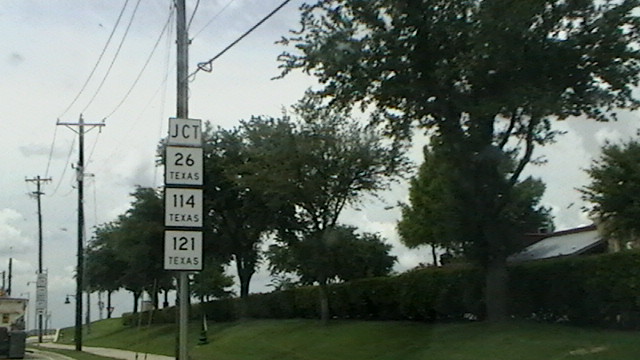In this outdoor color photograph captured on a sunny day with scattered clouds, the foreground showcases a lush green lawn leading up to a well-maintained hedge of vibrant shrubs. Just beyond the hedge, the rooftop of a house peeks through, flanked by surrounding trees. Dominating the scene, three gray metal power line poles stand prominently in the foreground, with visible power lines stretching across the sky. Attached to the most prominent power pole are four white, square signs with black lettering. The top sign reads "JCT" indicating a junction, followed by "26 TEXAS" in bold, all-caps text. Below that, another sign states "114 TEXAS," and the bottom sign displays "121 TEXAS." The organized arrangement of the signs suggests nearby route numbers, while the overall composition captures a serene suburban setting.